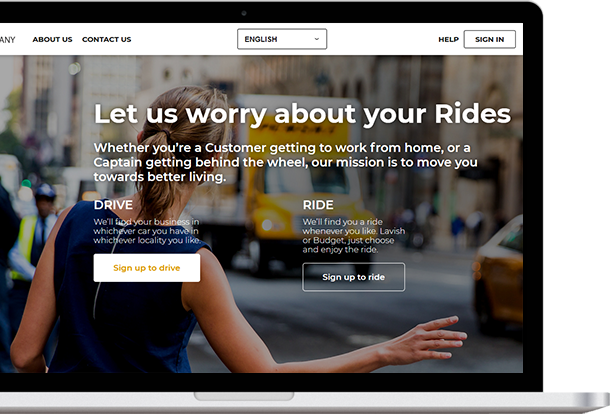### Descriptive Caption:

The image captures a partial view of a computer screen, with the left side slightly cut off. Dominating the screen is the front of a laptop, showcasing the top edge of the keyboard area and the black frame surrounding the screen. Along the top border of the screen, a white banner features navigation links in capital letters: "ABOUT US" and "CONTACT US." A drop-down menu nearby allows the user to select the language, currently set to English. On the far right, the banner includes a "SIGN IN" button and another button labeled "HELP."

Below the banner, the main visual element is a photograph of a woman in a blue dress, her back facing the viewer. Her brown ponytail is clearly visible as she raises her hand, seemingly trying to wave down a ride. The background showcases a blurred cityscape, emphasizing her action in the foreground.

The screen displays a prominent title in large font that reads, "Let Us Worry About Your Rides." Beneath this header, a smaller white text elaborates: "Whether You're a Customer Getting to Work from Home or a Captain Getting Behind the Wheel, Our Mission is to Move You Towards Better Living."

Further down, the screen is divided into two sections: one for drivers and one for riders. The driver section includes a "DRIVE" button, accompanied by text that states, "We'll Find Your Business in Whichever Car You Have in Whichever Locality You Like." A call-to-action button beneath it encourages users to "SIGN TO DRIVE" in yellow text on a white background.

Next to it, the rider section features the word "RIDE," followed by the text: "We'll Find Your Ride Whenever You Like, Lavish or Budget, Just Choose and Enjoy the Ride." This section also has a clear call-to-action button that reads "SIGN UP TO RIDE."

This detailed interface aims to cater to both potential riders and drivers, emphasizing convenience and personalized service.